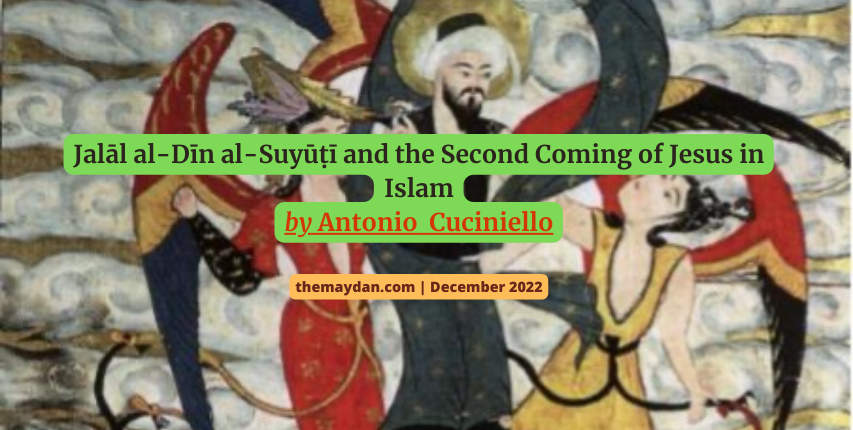The image is a colorful illustration, predominantly in white, gold, red, black, and silver hues, that is wider than it is long. It appears as a religious-themed artwork. The central figure is a bearded man wearing a turban topped by a black pillbox hat, dressed in a long black coat, and flanked by two women. The woman on the left is in a long red dress adorned with feathers in her hair, while the woman on the right wears a gold short-sleeved dress with a V-neck and has her hair styled in a black bun. All three figures have wings, which are black, gold, and red, creating ambiguity about their origin or to whom they belong. The backdrop resembles a white wall with cloud-like illustrations, contributing to the ethereal quality of the scene.

There is text prominently displayed on a green banner across the image, reading "Jalal al-Din al-Suyuti and the Second Coming of Jesus in Islam." Below this, in red letters, it says "by Antonio Guccinello." Additionally, a peachy orange box with brown lettering at the bottom of the image indicates "TheMaidan.com December 2022."